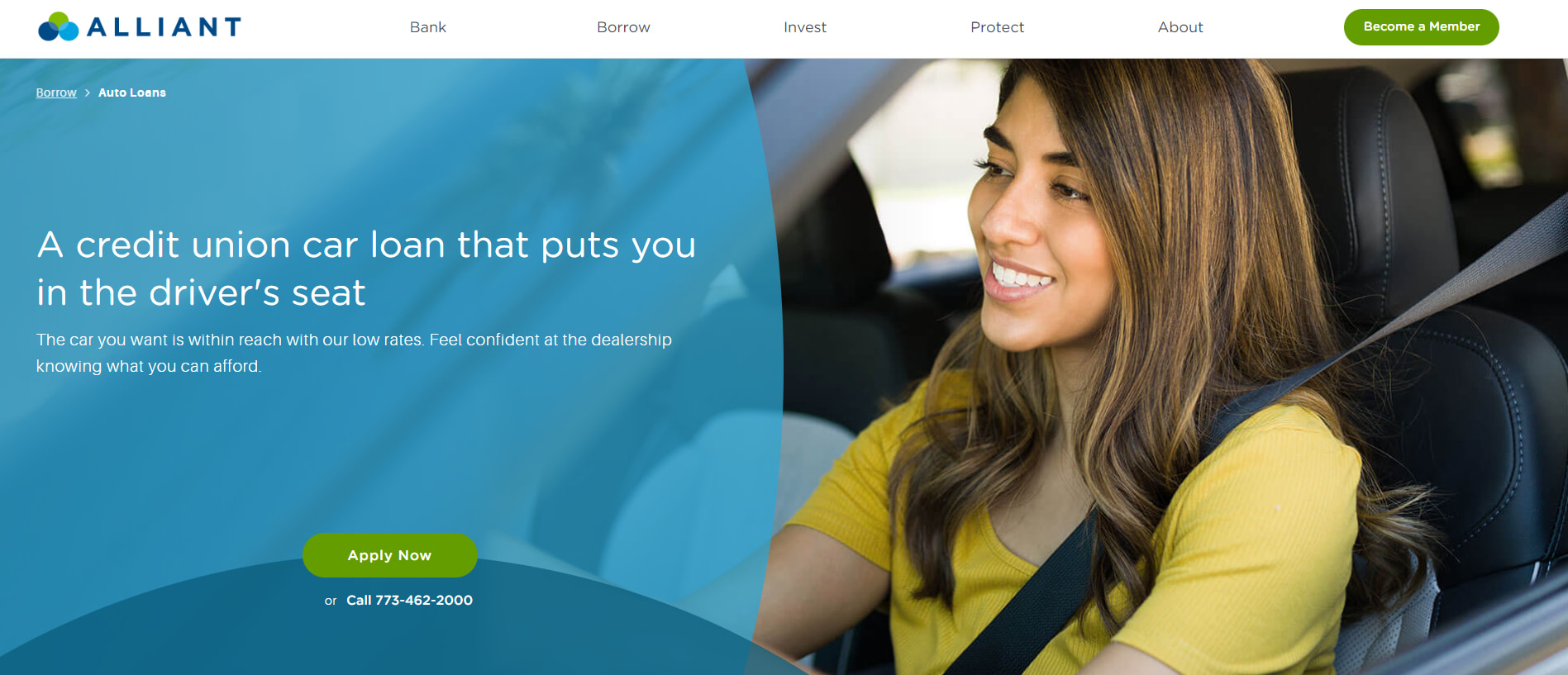Screenshot of Alliant Website - Banking and Investment Services

This screenshot captures the homepage of Alliant's banking and investment website, prominently showcasing their services and features. The Alliant logo, depicted in shades of blue and green, features two blue spheres (one dark, one light) supporting a green sphere, creating a visually appealing trio atop a white background.

The navigation bar at the top is clearly laid out with black text on a white background and includes the options: Bank, Borrow, Invest, Protect, About, and a prominent green oval button with white text that reads "Become a Member."

Centered on the page is an image of a woman with slightly tanned skin, wearing a cheerful yellow shirt. She is behind the wheel of a car or truck, smiling as she drives.

Adjacent to her image, a semi-transparent blue menu offers details about borrowing options, specifically focusing on auto loans. The text emphasizes the benefits of financing a car through Alliant credit union, highlighting low rates, confidence at the dealership, and affordability. This section includes a call-to-action with a green "Apply Now" button in white text and an alternative contact option, displaying the phone number 773-462-2000.

At the bottom, a darker blue semi-circle completes the design, reinforcing the website's focus on auto loans and showcasing Alliant's effort to promote their car loan services.